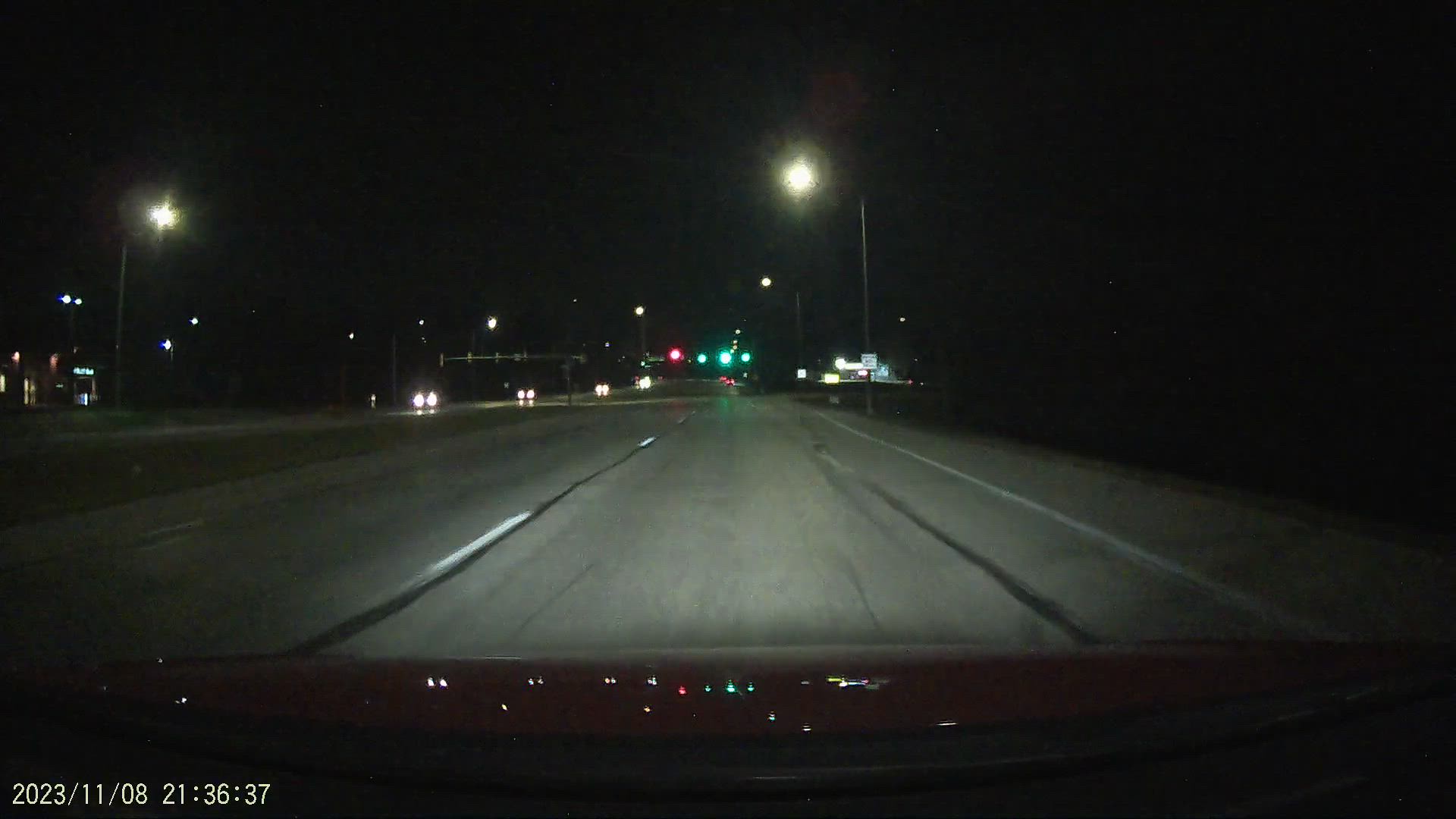A nighttime driving scene captured from a dash cam, showing the front windshield view of a car with a burgundy red hood. The car's headlights brightly illuminate the gray paved road ahead, revealing a lighter section of road compared to the darker distance. The road appears to have two lanes in the direction the car is traveling. Streetlights cast a faint white glow along the sides of the road, though most of the background is shrouded in darkness. In the distance, traffic signals are visible, with one red light on the far left and three green lights further ahead. The bottom left corner of the image features a date and time stamp reading "2023/11/08 21:36:37."